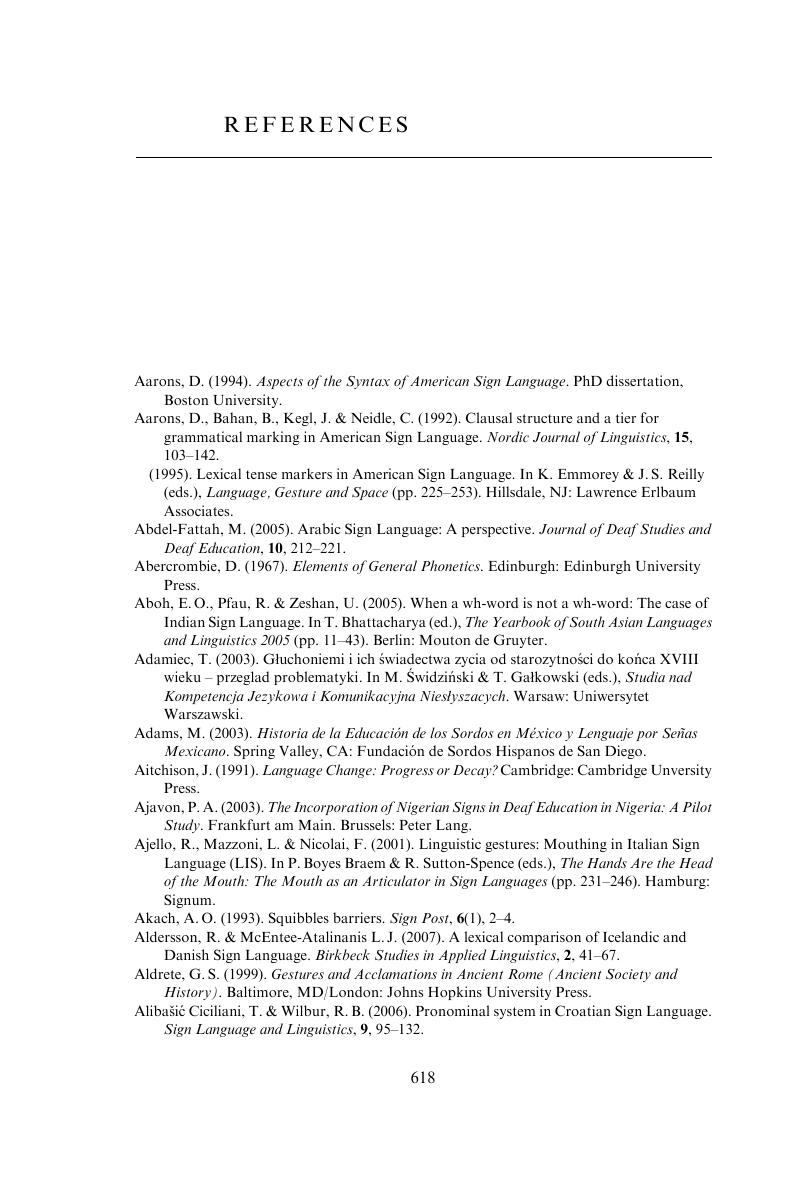The image depicts a reference page from a book, set against a white background with black text. At the top of the page, slightly offset to the left, the word "References" is prominently displayed. Directly beneath it lies a horizontal line followed by a considerable blank white space, equivalent to about the length of a paragraph. Under this white space, a list of references begins. The list includes approximately 11 to 12 entries, though the small print and slight blurriness make them difficult to read. The first entry is "Aarons, D. 1994. Aspects of the Syntax of American Sign Language, Ph.D. Dissertation, Boston University." This page serves as a comprehensive bibliography, indicating sources referenced throughout the book. The references cover various topics related to sign language and deaf communication, including American Sign Language, Nigerian signs in deaf education, linguistic gestures, and mouthing in Italian Sign Language. Situated at the very bottom of the page is the page number, 618.